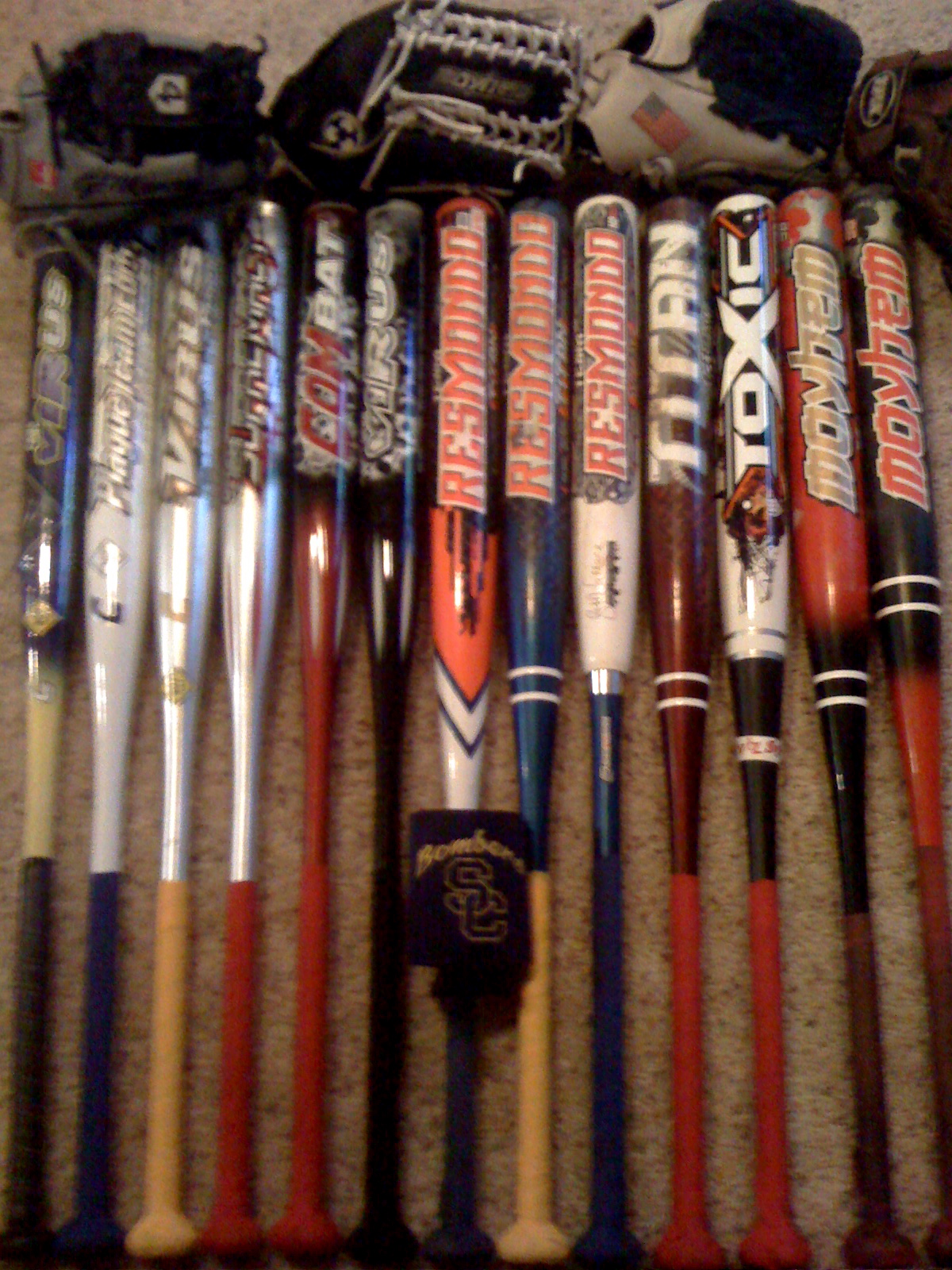This detailed photograph, taken indoors on beige carpet, showcases an extensive baseball collection meticulously arranged in a horizontal row. The collection features 13 aluminum baseball bats, each touching the next, creating a uniform layout. The bats exhibit a variety of colors and brand names, such as Resmondo, Titan, Toxic, Combat, and Mayhem, delivering a vivid spectrum from chrome and red to black, blue, and silver. At least three bats clearly display the brand Resmondo along their lengths.

Above the bats, aligned at their tips, are four baseball gloves: a black glove with white stitching, a white glove with black stitching and an American flag, a brown glove, and another in grey and black with a "4" on it. The photograph, while somewhat blurry and granulated in sections, also includes a brown or black can koozie marked "Bomberg SC" on the central bat. Additionally, some other indistinguishable sports equipment and a faint image of a baseball player can be seen in the background. The arrangement suggests a dedicated display, possibly in a custom-designed cabinet or case with a soft felt lining.